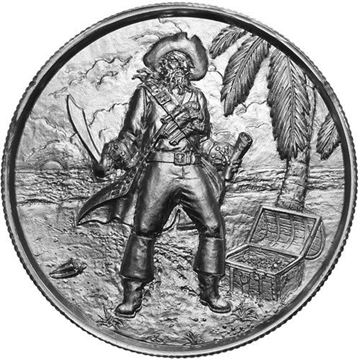The image features a large, round metal object resembling a coin, occupying the entire photo with a plain white background. The coin-like object, sculpted in various shades of grey and possibly some silver, showcases an intricately detailed scene. At the center stands a bearded pirate adorned with a hat, bandolier belt, and knee-high boots. He holds a sword in his right hand and a telescope in his left hand, not a map. To the right of the pirate, there's a treasure chest nestled beside a palm tree, with the shoreline and ocean visible in the background. The setting sun casts shadows, accentuating the pirate's rugged stance. Above the horizon, clouds drift lightly in the sky. The coin-like object, ridged along its edges, has no numerical or textual markings to denote monetary value, suggesting it might be a collectible or souvenir rather than actual currency.